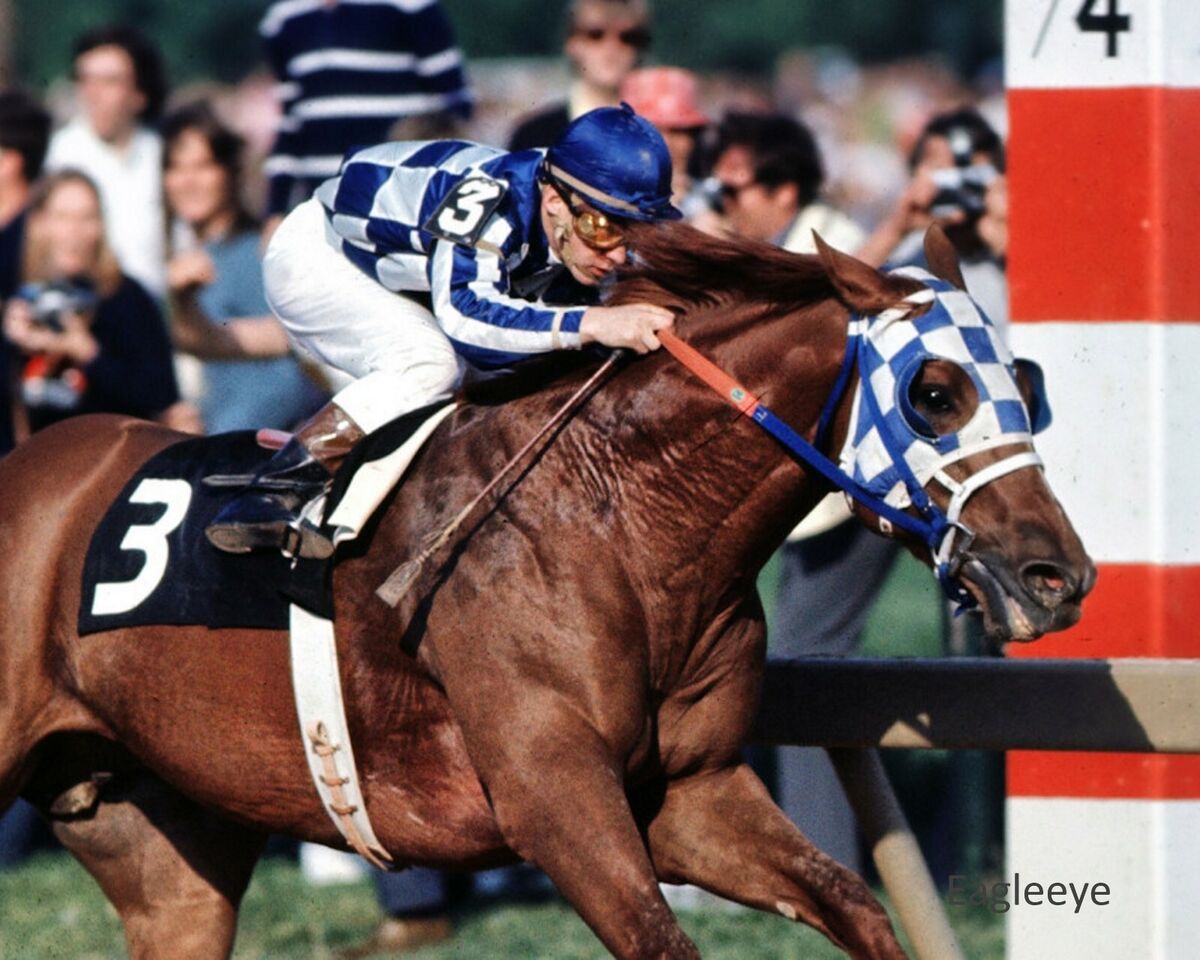This detailed still life captures the intensity and motion of a horse race, likely from an event such as the Kentucky Derby. The focal point is a jockey dressed in a blue and white checkered shirt, a blue cap, and white riding pants, all accented with black riding boots and goggles. Both the jockey and the brown, muscular horse he rides sport the prominent number three, visible on the jockey’s shoulder pad and the horse's black blanket. The horse also wears a matching blue and white checkered face mask and blue harness.

The background of the image shows a blurred crowd of spectators, some smiling and capturing the moment with cameras, emphasizing the photo’s focus on the subjects in motion. Among the spectators is a distinctive red, white, and blue pillar marked with the number four. The horse appears to be racing at significant speed, indicated by the lather on its coat and the jockey's crouched, focused position, likely using a whip for urging the horse forward. This photograph, taken in daylight at a racetrack, features a signature "D. Galea," suggesting the photographer who captured this dynamic and vivid scene.